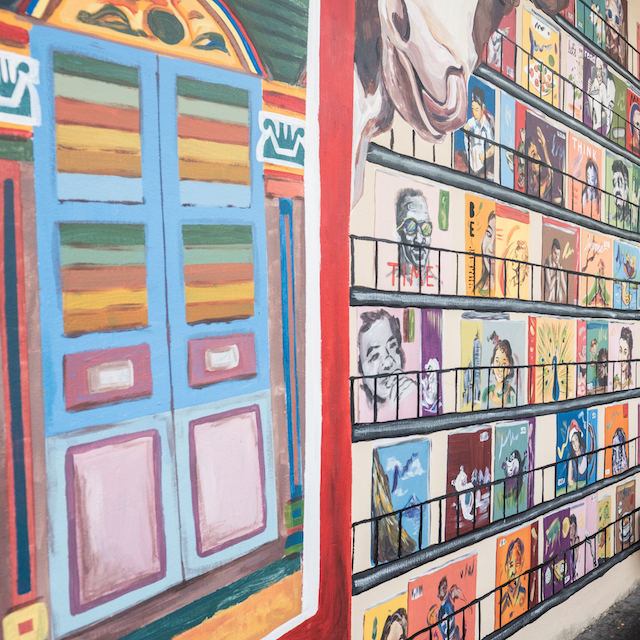The image showcases a vibrant mural bursting with multiple colors, possibly adorning the side of a building and featuring an intricate, Jamaican-inspired design. Dominating the left side of the mural is a painted wooden door, adorned with multiple panels in an array of dark green, light green, red, yellow, brown, and very light blue hues. Each panel is identically colored, with a pair of horizontal shapes and central white handles, adding a touch of realism. Right beside the door, painted shelves are stacked in at least six layers, supported by black rails. These shelves are filled with square items that are reminiscent of either books, CDs, or various cover images—some resembling Time Magazine covers, others suggestive of album covers, with each featuring different human figures. Adding a whimsical element, the top right corner of the mural displays a partial image of a cow with its tongue playfully sticking out. The cow's nose and neck stand out, providing a quirky touch to the multi-colored artwork.